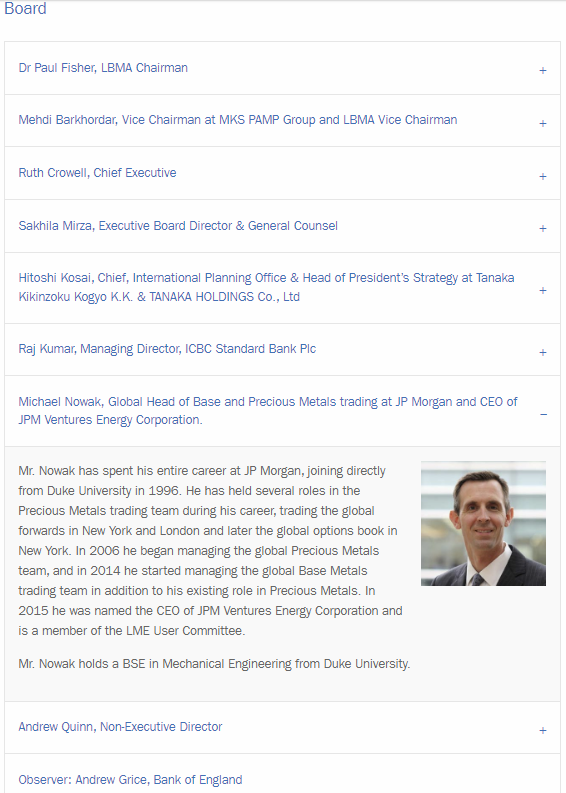This image appears to be a screenshot captured either from a phone or a computer screen, displaying an organized listing of board members. At the very top left corner, in blue text, it says "Board". Below this heading, the board members' names and titles are listed in a drop-down format, with a total of eight main entries and additional options at the bottom.

1. **Dr. Paul Fisher** - LBMA Chairman.
2. **Middy Barkorder** - Vice Chairman at MKSPAMP Group and LBMA Vice President.
3. **Ruth Crowell** - Chief Executive.
4. **Sakhila Meza** - Executive Board Director and General Counsel.
5. **Hitoshi Kosai** - Chief International Planning Officer and Head of President Strategy at TANQA, Kizoku, Koyo, KK, and Tonka Holdings.
6. **Raj Kumar** - Managing Director, ICBIC Standard Bank.
7. **Michael Nowak** - Global Head of Base and Precious Metals Training at JP Morgan and CEO of JPM Ventures Energy Corporation.

Additionally, there is a paragraph that appears to provide a detailed description of Mr. Nowak. Below this list, there are two more choices:

8. **Andrew Quinn** - Non-Executive Director.
9. **Andrew Grice** - Observer from the Bank of England.